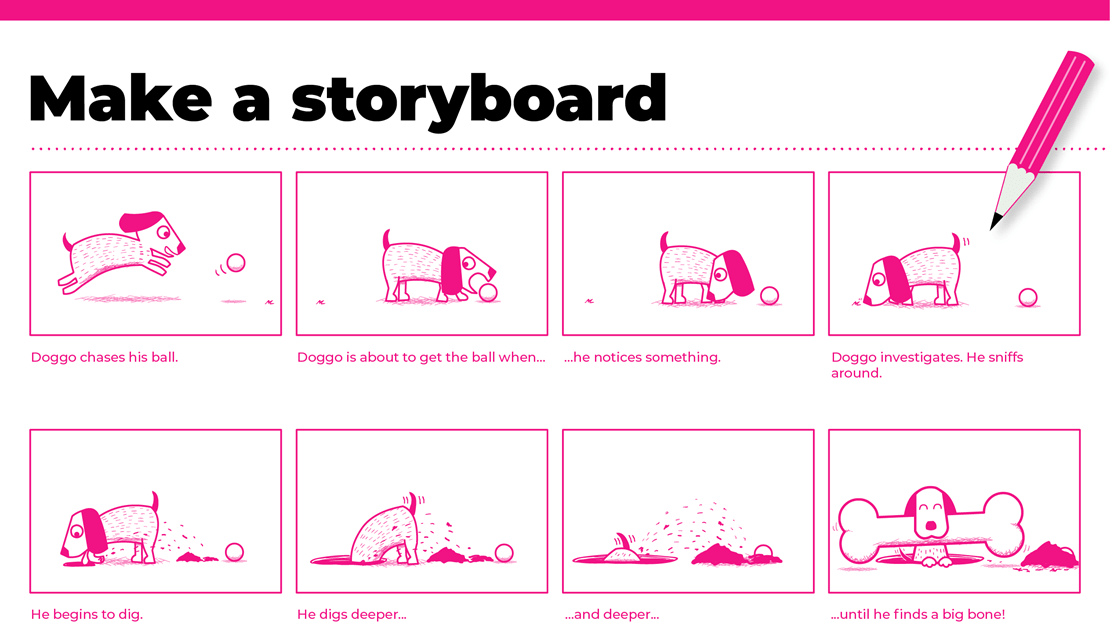This illustration serves as an example of how to create a storyboard, dominated by a pink and white color palette. At the top, a hot pink bar caps the image, followed by the bold black text "make a storyboard." Directly below this, a dotted pink line divides the header from the main content. The storyboard consists of eight pink-framed rectangles, each containing a pink illustration of a dog named Doggo in various actions. The scenes, each accompanied by descriptive text, start with "Doggo chases his ball," then "Doggo is about to get the ball when..." leading to "he notices something." Following these, Doggo "investigates" and is depicted sniffing around. Next, "he begins to dig," with subsequent frames showing Doggo digging progressively deeper ("he digs deeper" and "and deeper") until the final frame where "he finds a big bone," showing Doggo with a large bone in his mouth. In the top-right corner, a prominent pink pencil with black lead points diagonally downward toward the middle-bottom of the image.